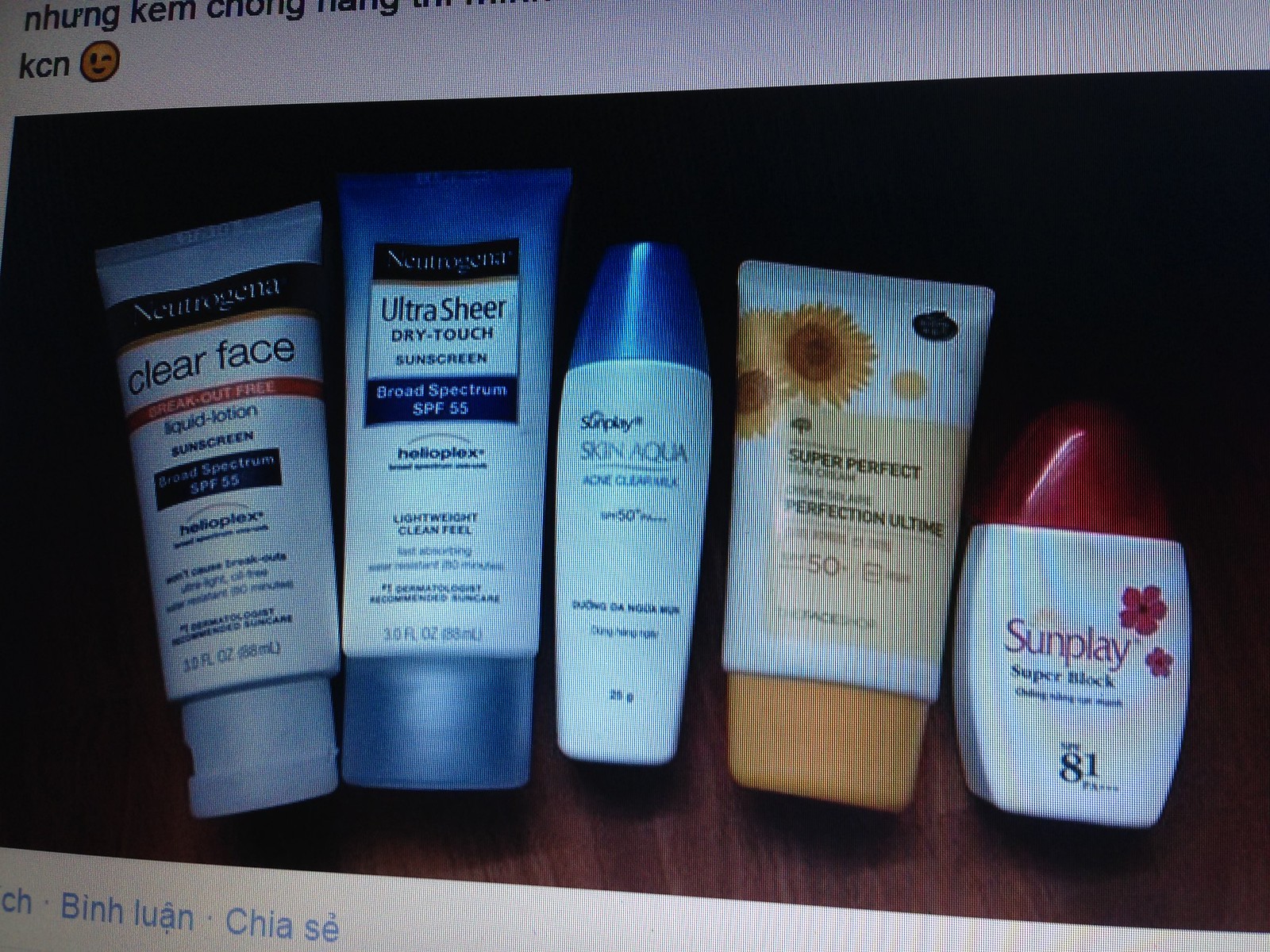The photograph, apparently captured of a digital magazine display, exhibits the distinct visual artifacts of swirls and lines caused by the screen's refresh rate. The main focus of the image is a row of five personal care products, predominantly sunscreens, from the brands Neutrogena and SunPlay, arranged from left to right. 

The first two products are from Neutrogena, featuring tube-shaped containers that identify themselves as "Clear Face Liquid Lotion" and "Ultra Sheer Dry Touch," both largely white with black text accents. The adjacent SunPlay products exhibit a variety of colors: one has a white body with a blue cap, likely a roll-on deodorant; another displays white packaging adorned with sunflowers and a yellow cap. The final product on the far right, also from SunPlay, has a white body topped with a red triangular cap. 

The text in the image includes English and an indeterminate Asian language, possibly Thai, suggesting the photograph might be from an international magazine ad. The SPFs of these products range from 50 to 81, indicating various strengths and formulations.